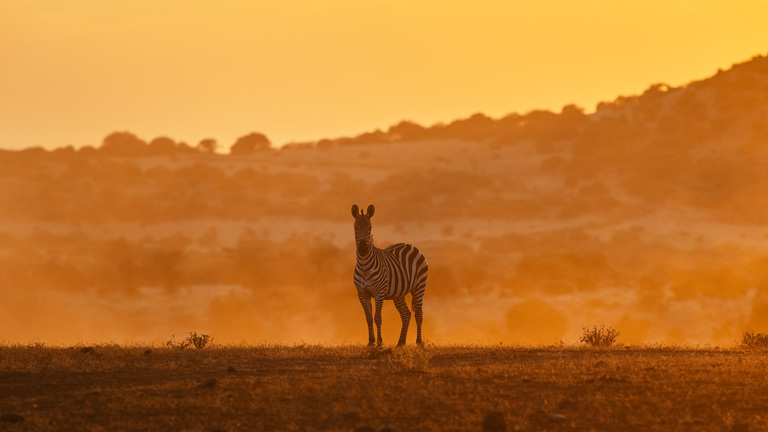In the warm, orange-hued photograph, a zebra stands prominently in the middle of a flat, grassy savannah, appearing almost as if poised on a perfectly level shelf that occupies the bottom one-sixth of the image. The zebra is facing the camera, its body slightly angled so that its rear tilts to the right and its front towards the upper left. Behind the zebra, the landscape transitions into gently sloping, brush-covered hills which fade into deeper shades of orange and brown under the same pervasive golden lighting. The horizon line sits about one-third from the top of the image, merging the flat grassland with the elevated terrain in the background. Above this, the sky glows in a yellowish-orange tint, completing the scene's cohesive, sun-drenched ambiance.